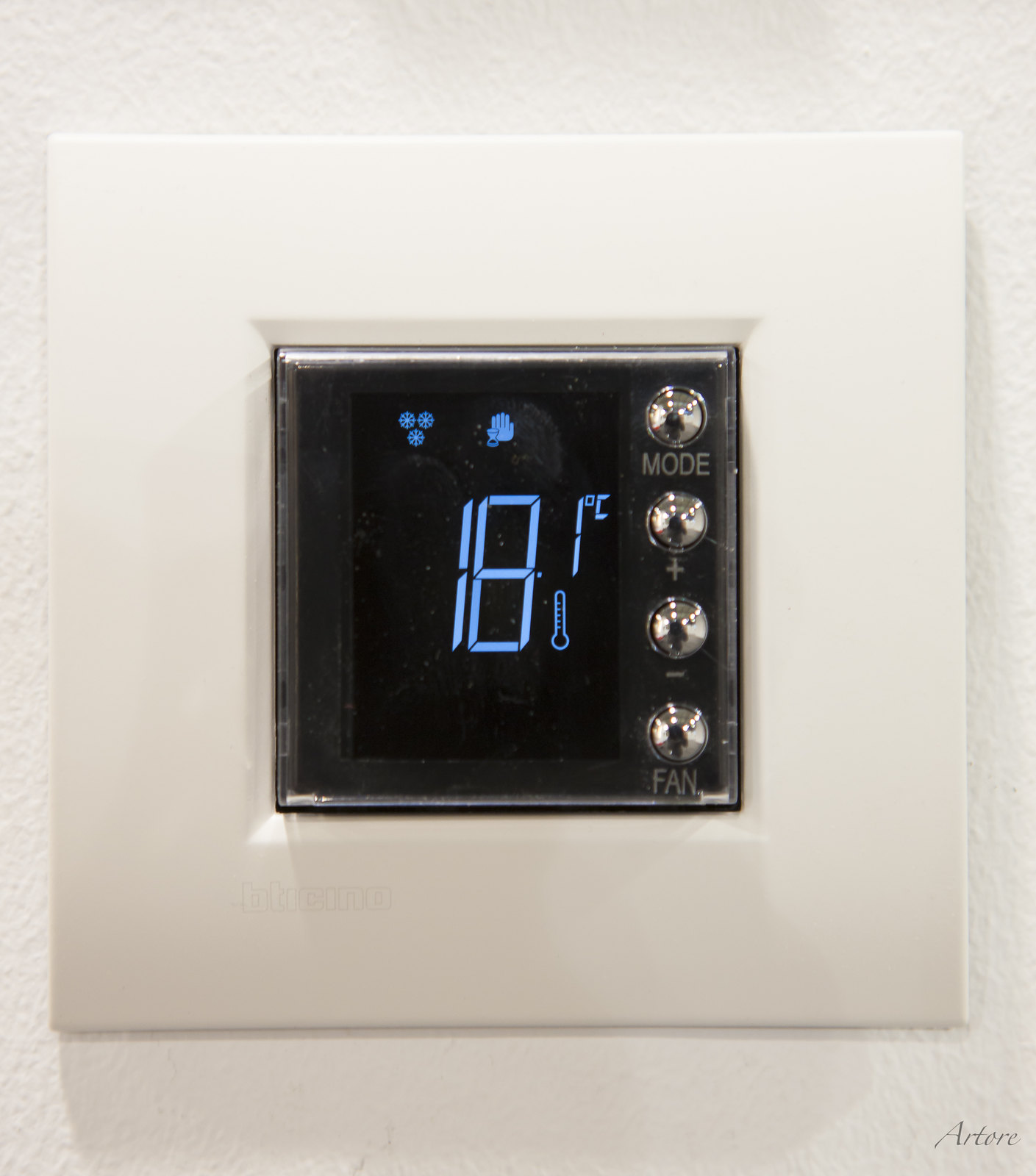The image depicts a thermostat mounted on a textured white wall, photographed indoors with a regular camera. The wall's texture and the slight color variation between the wall and the thermostat are noticeable due to the shadowing caused by the ambient light, which creates a subtle outline around the device. 

In the lower corner of the wall, the word "ARTERO" is visible, although the spelling might be "ARTROR" or "ARTROE." The thermostat itself features a large, white, square frame that encompasses a smaller, central black digital display. 

The thermostat reads 18.1 degrees Celsius and includes a thermometer icon with a bulb at the bottom that extends upward. The top left corner of the screen displays three small circles adjacent to a vague bluish shape. Along the right side of the thermostat are four vertically aligned buttons: the top one labeled "Mode," followed by a plus sign, then a minus sign, and the bottom button marked with a fan symbol.